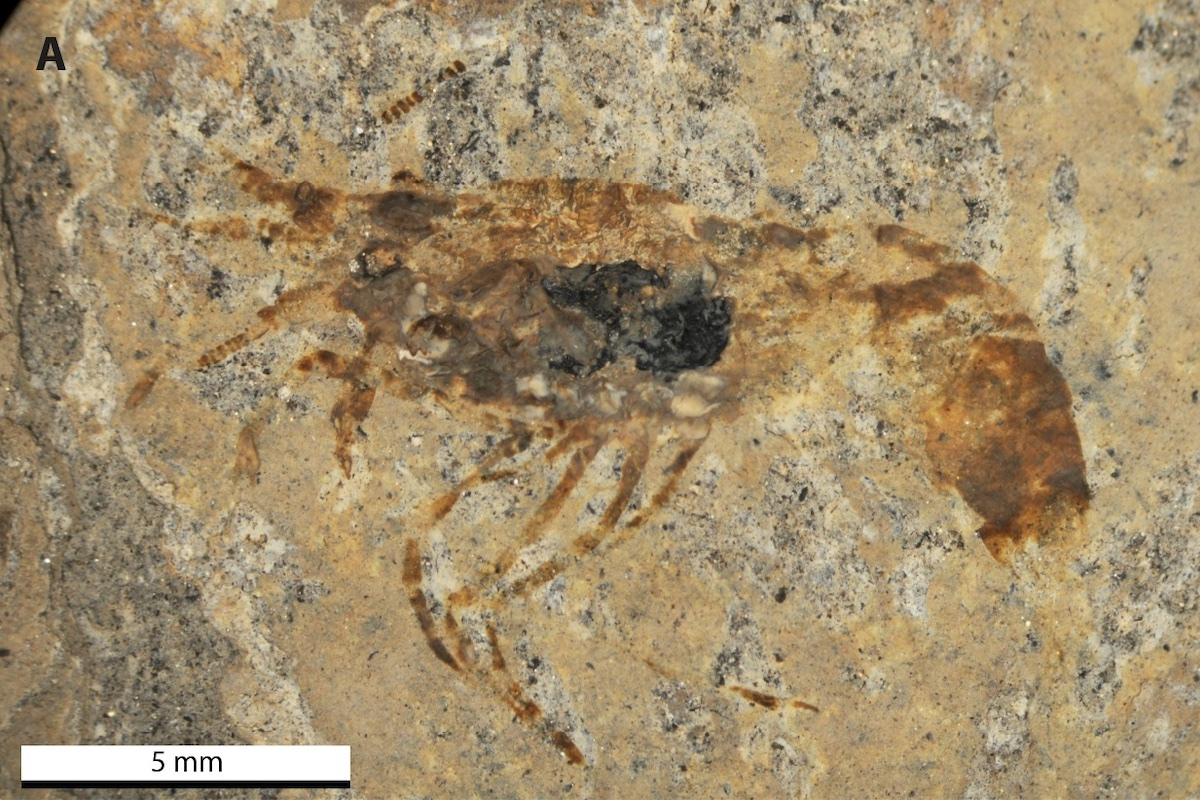This image captures a close-up of a gray rock surface featuring a detailed, fossil-like imprint that appears to depict an ancient creature, possibly resembling a shrimp, bird, or insect. The imprint, prominently located in the center of the photograph, exhibits a rich, rusty brown color with areas of darker, almost black markings, suggestive of areas where the organism likely decomposed, leaving behind a textured stain. The overall composition of the imprint includes identifiable features such as a head, body, and appendages resembling legs, enhancing its plausibility as a fossil. Additionally, in the bottom left corner of the image, there is a clear, white rectangle containing the notation "5mm," which provides a sense of scale. The rock texture around the imprint is rough and gray with scattered stains, indicating weathering and age, reinforcing the ancient and possibly prehistoric nature of the imprint.